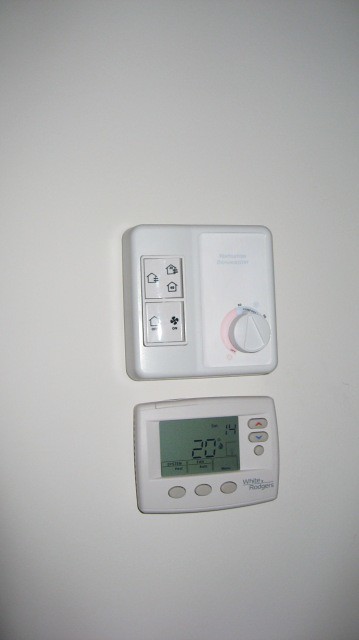The photo presents a minimalist scene featuring two white thermostats mounted vertically on a pristine white wall, designed for home temperature regulation. The upper thermostat, a larger, perfectly square device, boasts a simple interface with two square buttons aligned vertically on the left side. The top button, adorned with three distinct house icons, likely manages various home temperature settings. Below it, a button displaying a house and a fan symbol appears to control the house fan. Adjacent to these buttons is a rectangular panel with a single knob that allows users to adjust the temperature—hotter to the left and cooler to the right.

Beneath this mechanical thermostat, a more modern, digital counterpart takes its place. This smaller, sleek device features a centered screen that clearly displays the current temperature at 20 degrees Celsius. It includes three gray buttons aligned horizontally below the screen and two vertical buttons positioned to the right, designed for precise temperature adjustments. This juxtaposition of analog and digital elements presents a comprehensive and user-friendly approach to managing home climate.